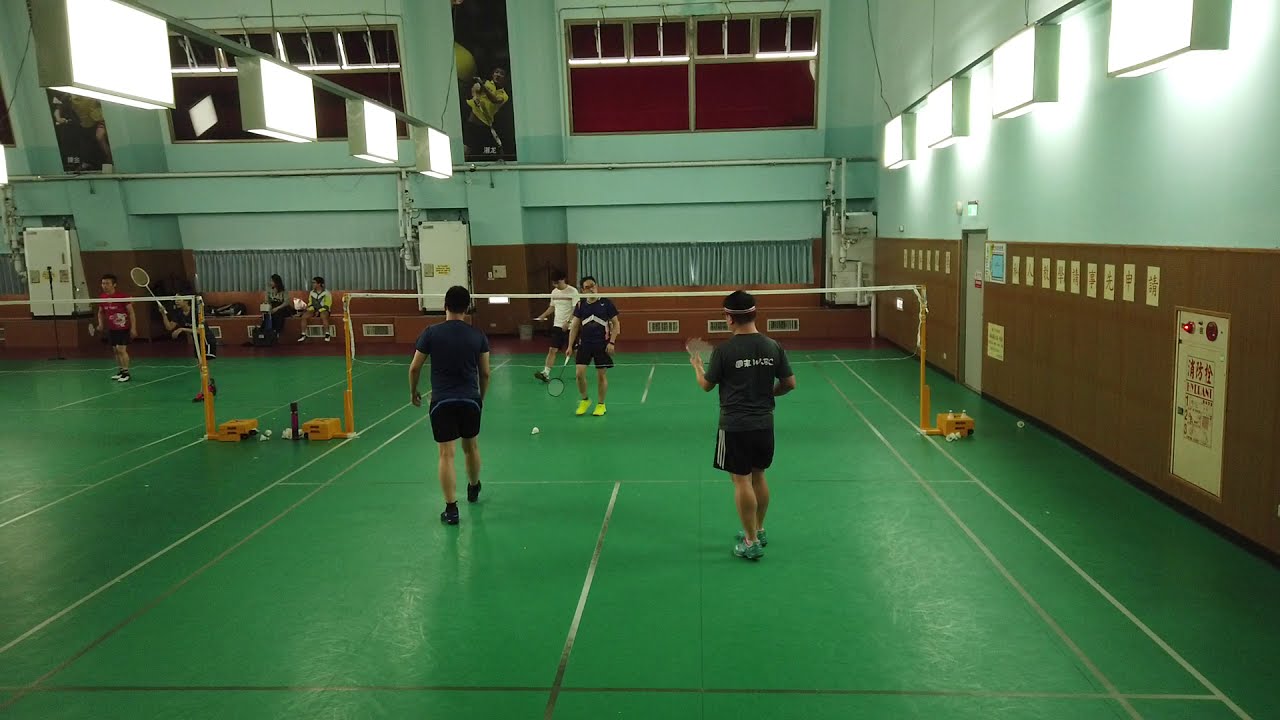The full-color, horizontally rectangular photograph depicts an indoor gymnasium setting. The gymnasium features white walls adorned with red areas and white trim, possibly indicating the presence of windows. The ceiling is lit by several square-shaped block lights. The green, smooth, hard flooring stretches across the scene, providing the stage for the ongoing activity.

Central to the image are two games of badminton, each with a white net supported by yellow posts. On both sides of the nets, two players are engaged in play, holding their badminton rackets. To the far left of the frame, part of another game is visible, along with a couple of spectators watching the matches. The color palette of the scene includes green, orange, black, gray, white, red, and silver, contributing to the lively and vibrant atmosphere of the indoor sports setting.